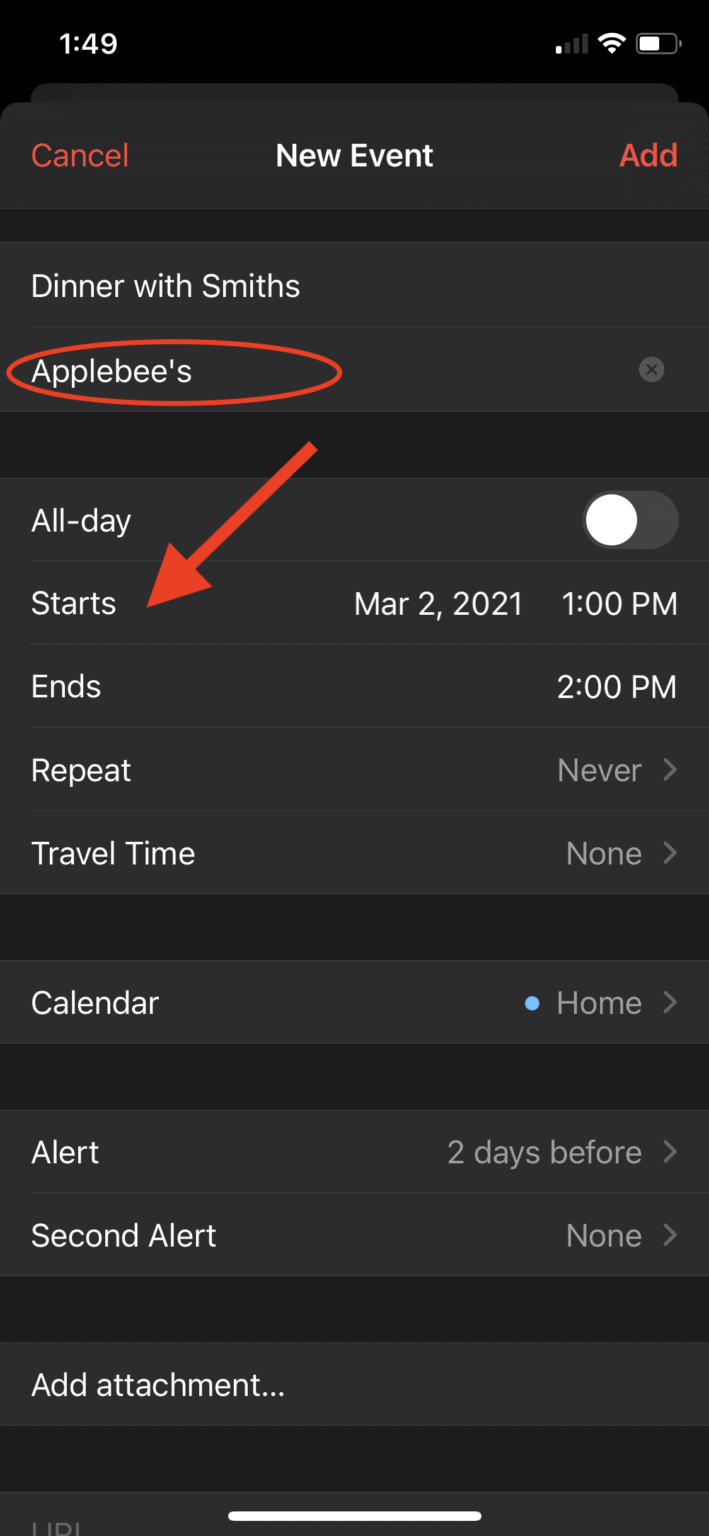An image shows a screenshot of a smartphone's calendar interface. The background is predominantly black. At the top left corner, the time is displayed as 1:49, with various icons to the right, including a battery icon that appears about two-thirds charged with a white line in the middle.

Beneath this top bar, the next section displays "Cancel" in red print on the left, "New Event" in white print in the center, and "Add" in red print on the right.

In the main part of the screen, the event title "Dinner with Smiths" is written in white text, followed by the location "Applebee's," also in white. "Applebee's" has been circled with a digitally added red oblong circle and a red arrow pointing downwards to the word "Starts."

Below this, the event start date and time are indicated as "March 2nd, 2021, 1:00 PM." Above the start time, "All-day" is listed with a slider that is currently in the off position.

Continuing downwards, white text displays additional event details sequentially as "Ends," "Repeat," "Travel Time," "Calendar," "Alert," "Second Alert," and "Add Attachment…"